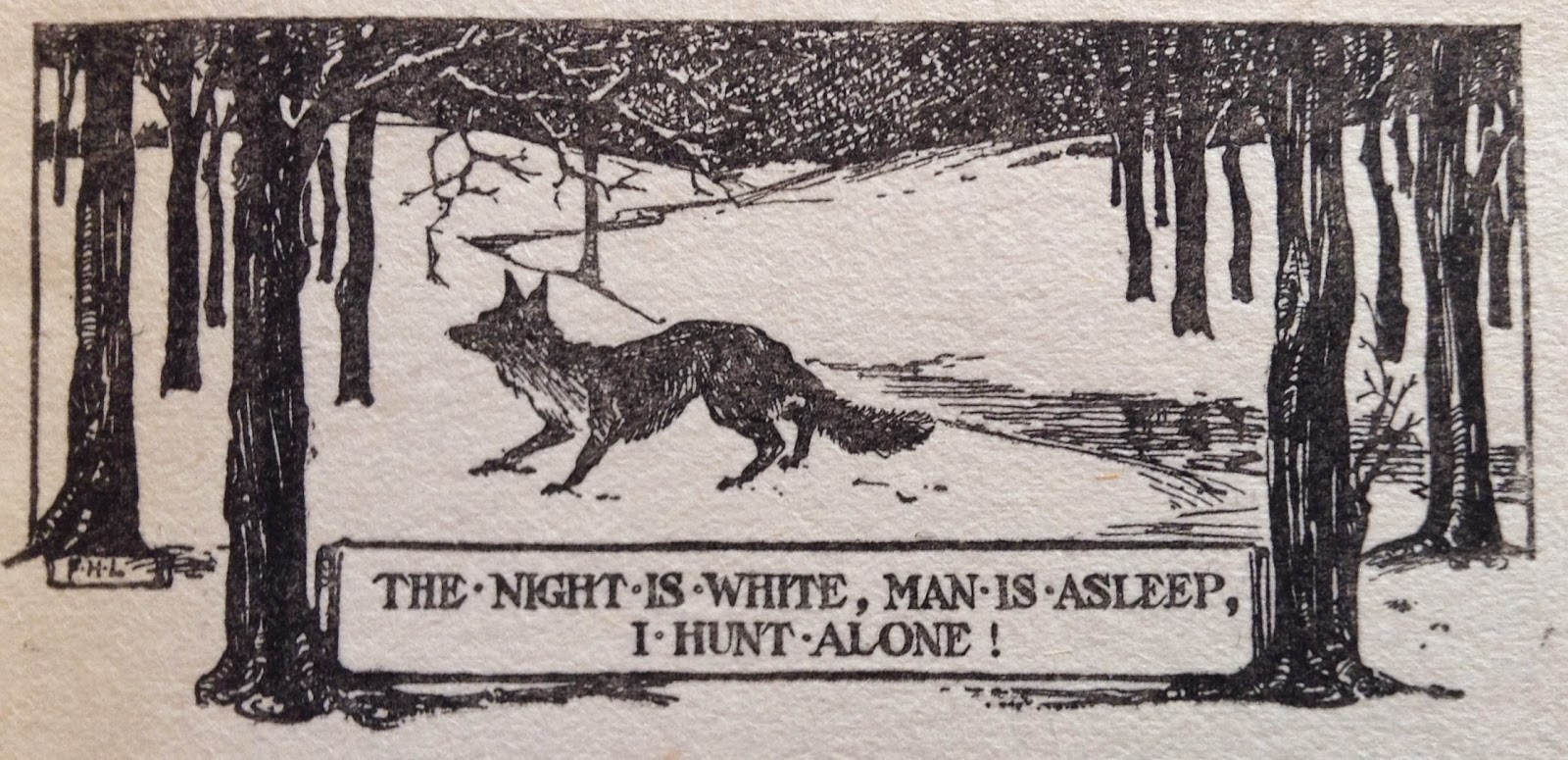This is a detailed black and white hand-drawn image of a fox moving from right to left through a snowy, leafless forest at night. The fox, predominantly black with a touch of white on its chest, is seen in its left profile, with its footprints trailing behind in the snow. The forest comprises about 15 barren trees and a faint hill in the background, which fades into the darkness, implying a nighttime setting with a black horizon. Snow covers the ground entirely, and we see some broken branches among the trees. At the bottom of the image, a white banner with black, all-capitalized text reads: "THE • NIGHT • IS • WHITE, MAN • IS • ASLEEP, I • HUNT • ALONE." This caption, possibly from the fox's perspective, underscores its solitary hunt in the quiet, snowy woods.